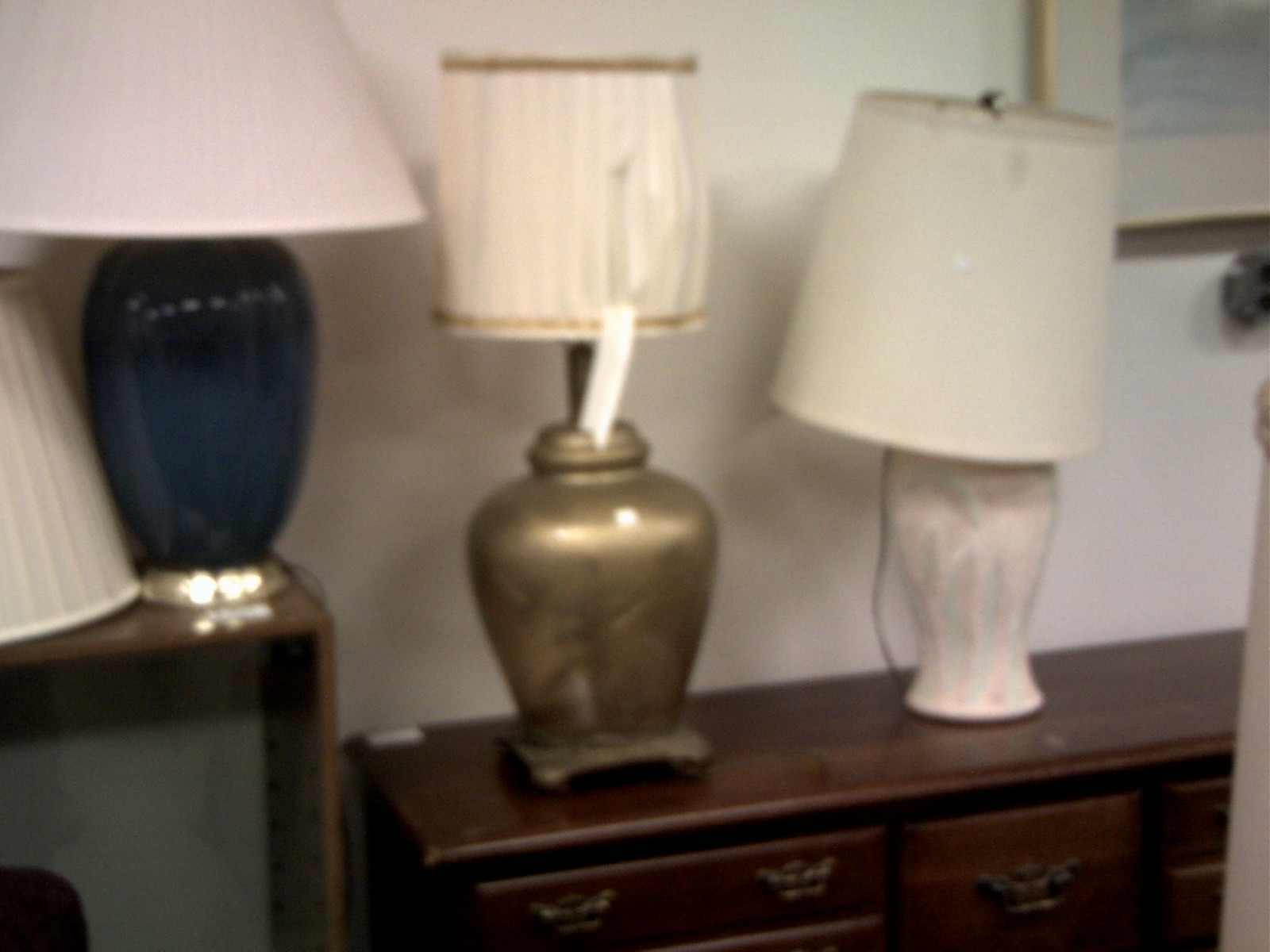In this somewhat blurry and out-of-focus photograph, the image captures an off-white, potentially white wall as the backdrop, with uneven lighting contributing to its off-color appearance. Positioned against the wall are two pieces of dark brown wooden furniture. To the left stands a taller table, which hosts a blue lamp with a white shade and another white lampshade to its left. The wider, long dresser extends to the right edge of the image and features several drawers adorned with older-style hardware. Atop this dresser are two more lamps: one with a gold base and a beige shade, and another with a slightly disheveled white shade and a white base, accompanied by a noticeable black cord. In the upper right corner of the photograph, the frame of a picture is faintly visible.